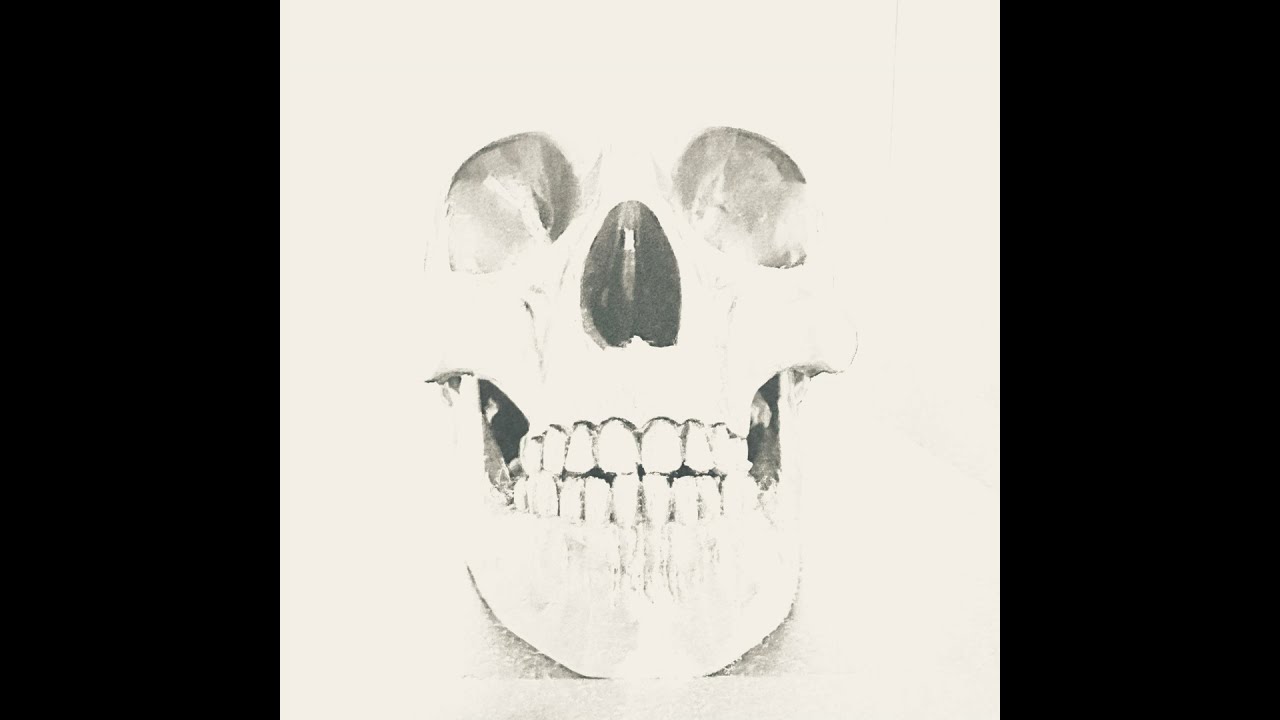This is a detailed, hand-drawn pencil sketch of a human skull, prominently displayed on an off-white, possibly beige sheet of paper. The artistic illustration, devoid of any text, sits against a stark black background, creating a dramatic contrast. The skull is centrally positioned within the image, facing directly toward the viewer, with detailed features such as the eye sockets, nasal cavity, jawline, and intact teeth clearly visible. The sketch highlights various shades of gray, blending into the background without a definitive outline, giving the impression of a "vanishing smile." The skull's periphery appears to dissolve into the paper, particularly at the top and sides, suggesting an overexposed or ethereal quality. This composition is flanked by thick black rectangles on both the left and right sides, which further emphasizes the central skull motif. The overall grayscale scheme and the black framing create a compelling, almost ghostly effect.